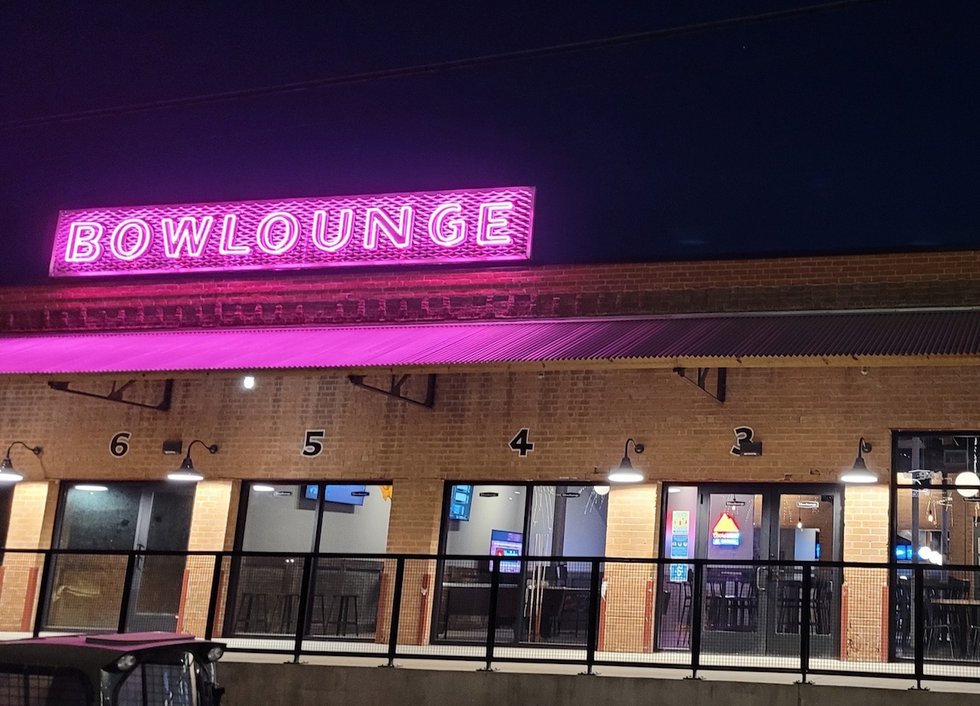This image captures a night scene outside a retro-themed bowling lounge named "Bowl Lounge," prominently displayed in vibrant pink neon lights on the left side of the single-story building. The building, made of yellow brick, appears to have been repurposed from an old loading dock, as indicated by the numbered windows and doors marked 3, 4, 5, 6. These rectangular windows with black frames offer a glimpse inside, revealing stools, tables, and pool tables, along with a number of TVs mounted on the walls. The exterior includes a wide concrete patio area bordered by a thin black metal railing. The dark night sky serves as a backdrop, with the neon sign's bright pink reflection illuminating the scene.